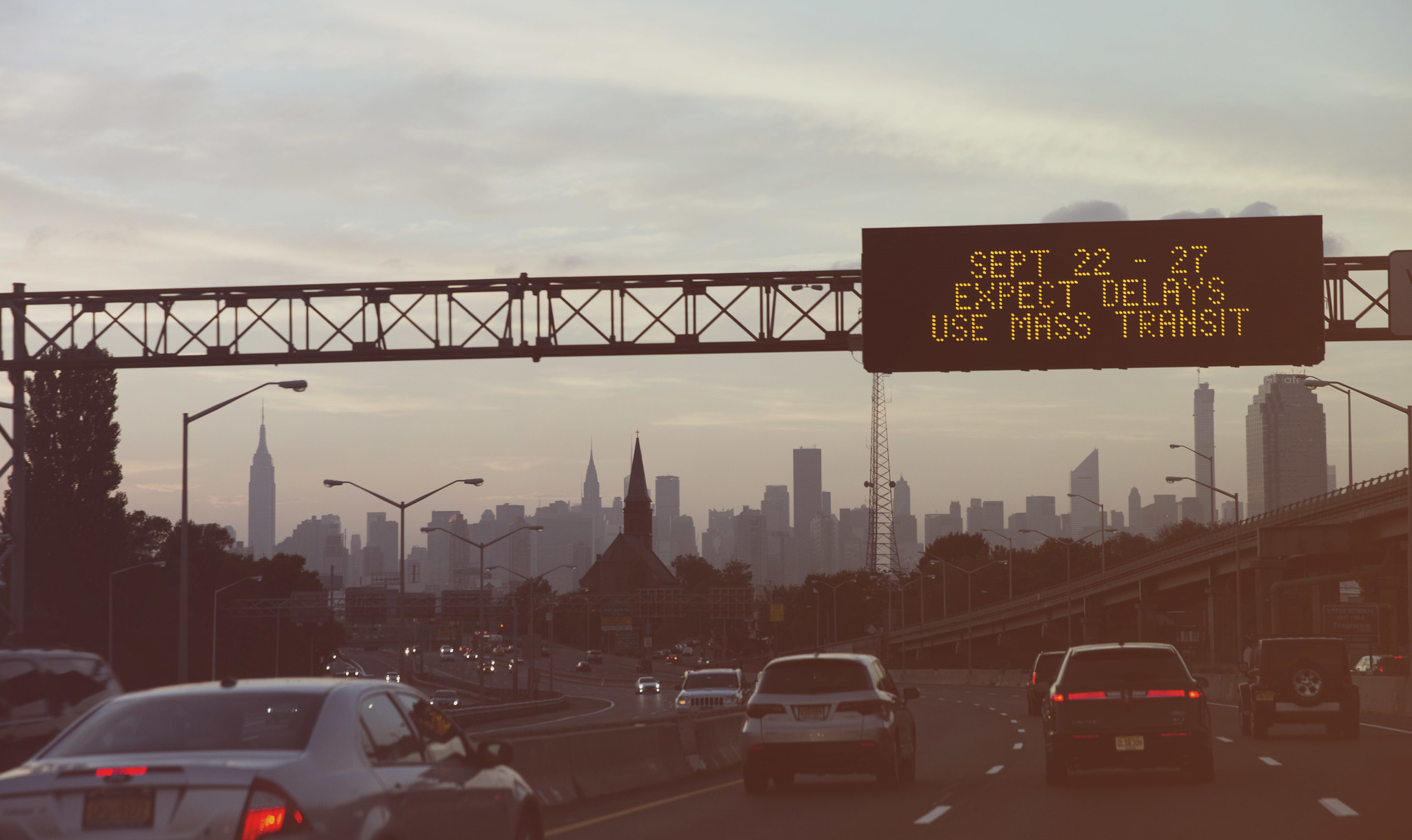This image captures a bustling street in what appears to be a major city, likely New York City or Chicago, evidenced by the tall high-rise buildings in the background that are silhouetted against a light blue and slightly gray sky. The immediate foreground showcases a traffic scene viewed from within a vehicle. There are three visible lanes of traffic directly in front, separated by a median to the left, which contains at least two additional lanes. A larger median separates this set of lanes from yet another section of road with more lanes, indicating a highly complex and busy urban road network. Overhead, a metal structure supports a digital information sign, which is black with yellow letters. The sign reads: "SEPT 22nd to the 27th 22-27 expect delays use mass transit," alerting drivers to upcoming traffic delays and encouraging the use of mass transit.